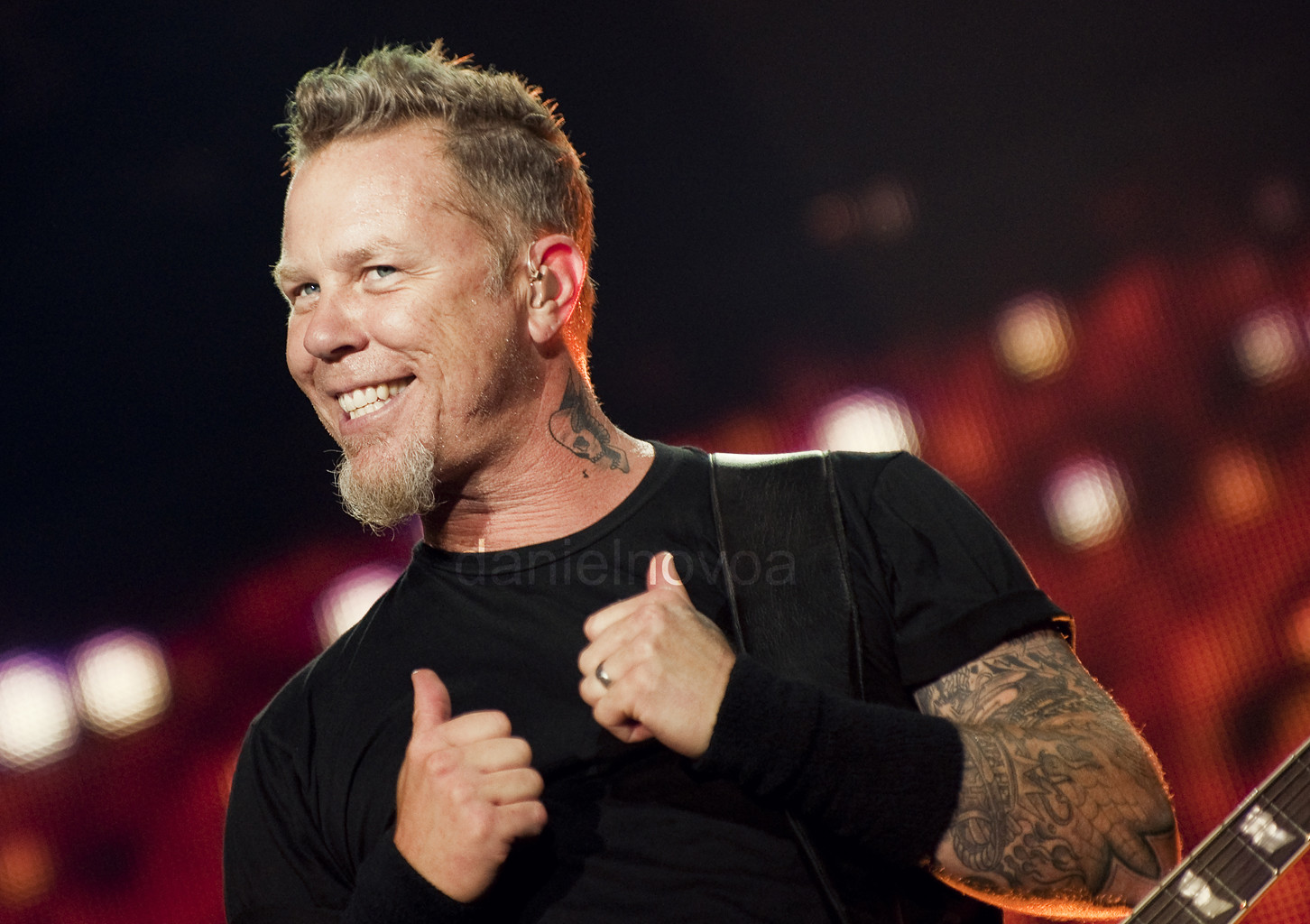The image features James Hetfield, a member of Metallica, standing at a concert. He is positioned in the middle of the frame with his head turned slightly to the right, smiling and looking off into the distance. He wears an earpiece typically used by performers, and he has a guitar strap over his shoulder, indicative of his readiness to play. His attire includes a short-sleeved black t-shirt, black wristbands, and a ring on his finger. Visible tattoos adorn his arms and neck. The background is highly blurred, consisting of stage lighting that creates a faded, multicolored ambiance with shades of black, beige, blonde, gray, red, white, and yellow. The prominent guitar shaft can be seen in front of him extending towards the bottom right corner of the image. The text over the image reads "Daniel Norwop," but this appears to be a mislabeling, as the individual is clearly James Hetfield.